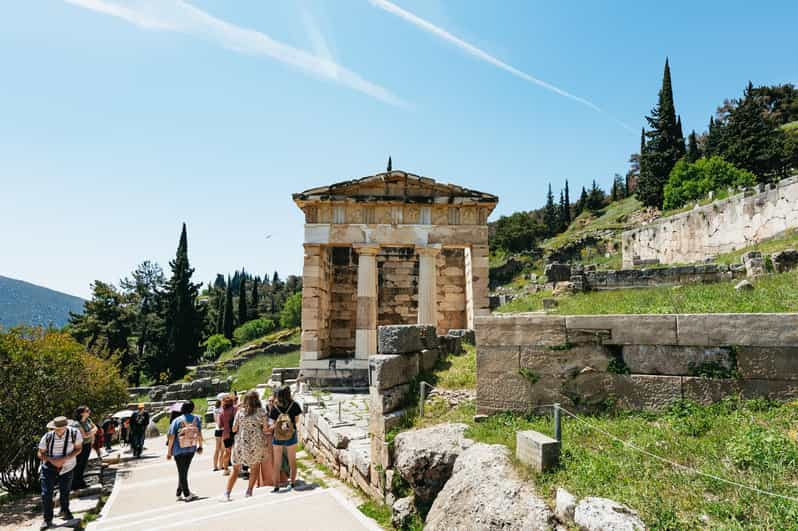This image captures a picturesque European ruin, likely located in the Mediterranean region, under a clear, blue sky crisscrossed by faint aeroplane contrails. Central to the photograph is an ancient stone temple, distinguished by its white stone construction and two prominent columns supporting a low, pointed roof. The temple occupies roughly a fifth of the image and features seven Roman numerals carved under the roof. In front of the temple, there's a triangular section of stone slabs and old walls extending outward. 

The scene is set on a terraced, hilly landscape -- the hill slopes upward from left to right at about a 35-degree incline. In the distance, coniferous trees dot the horizon. To the left, a modern stone wall, made of three layers of large, flat stones, complements the ancient architecture, extending from the bottom to the base of the temple. The foreground features a modern footpath with stairs, accommodating approximately 12 tourists, some of whom are climbing the steps, while others are observing the historical site. The visitors, identifiable by their backpacks and cameras, suggest that this ancient ruin is a popular tourist destination. Additional old stone walls and possibly another monument or a cemetery are discernible in the background, contributing to the area's historical ambiance.